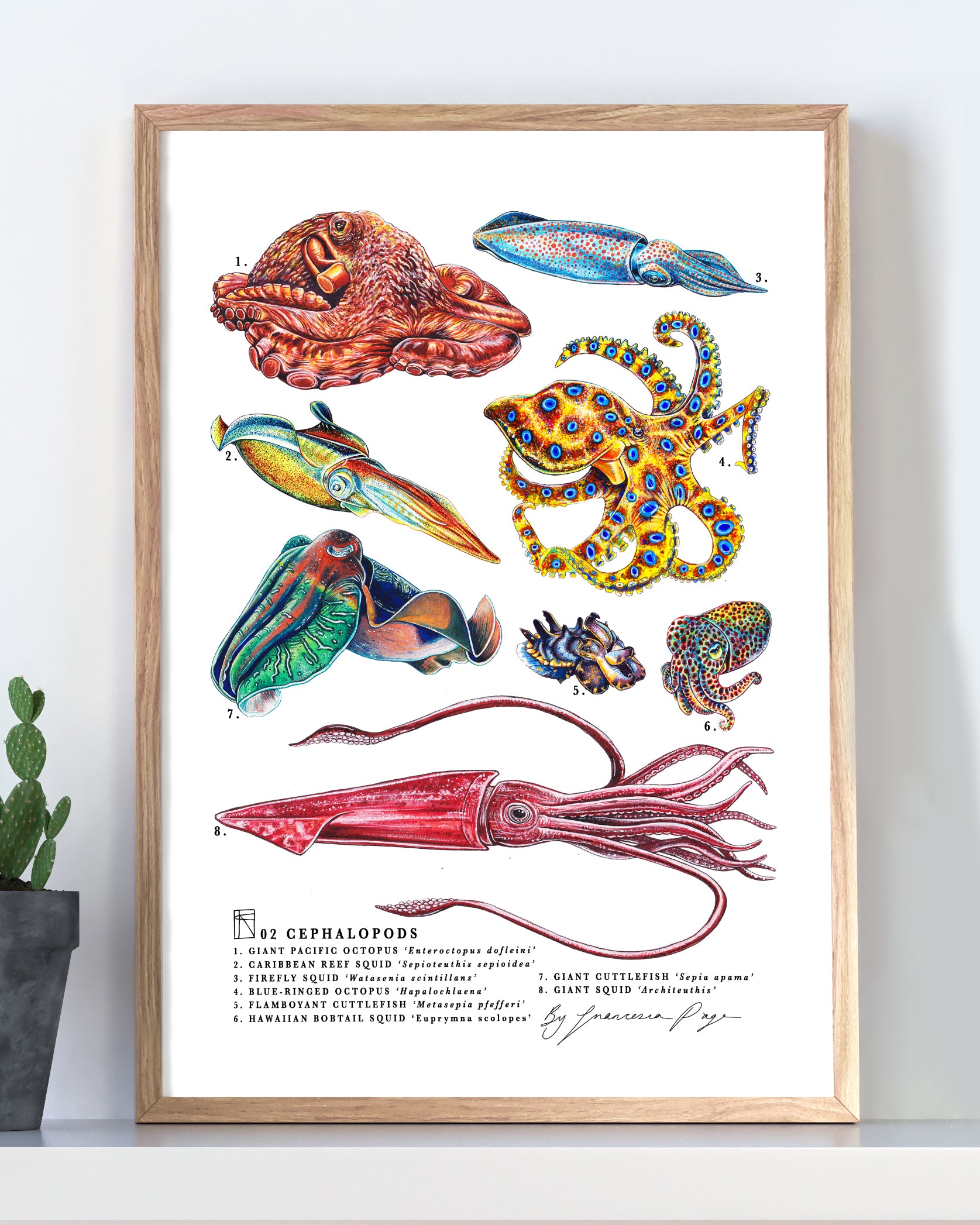This detailed photograph captures a framed scientific poster of cephalopods, elegantly displayed on a mantle. The poster, held in a plain tan wooden frame, stands next to a small green cactus in a gray ceramic pot. Its white background showcases eight distinct sea creatures, featuring a vivid palette of green, red, yellow, and blue. The creatures, including various species of octopuses, squid, and cuttlefish, are strategically numbered from 1 to 8, correlating to their names listed below in small, finely printed text that's somewhat difficult to read.

At the top of the poster, the red and orange-tinted giant Pacific octopus lays its head back, while next to it, the slender, blue-colored firefly squid, adorned with orange dots, captures attention. The yellow and blue-hued blue-ringed octopus, with its tentacles sprawled in a star pattern, adds to the vibrant display. The Caribbean reef squid, reminiscent of a duck with its orange, yellow, and blue tones, is placed to the left.

The lower section features the giant cuttlefish, displaying its blue alien-like body with greenish veins. Nearby, the flamboyant cuttlefish intrigues with its mix of blue and purple hues. The Hawaiian bobtail squid, a somewhat endearing creature with its bright green eyes and red spots, adds a touch of charm.

At the very bottom, the formidable giant squid, rendered in a striking red color, extends its tentacles dramatically, with one black eye seemingly gazing directly at the viewer. The detailed and methodical arrangement, accompanied by the Latin names of each species, makes this poster resemble a page from an antiquated botanical book.